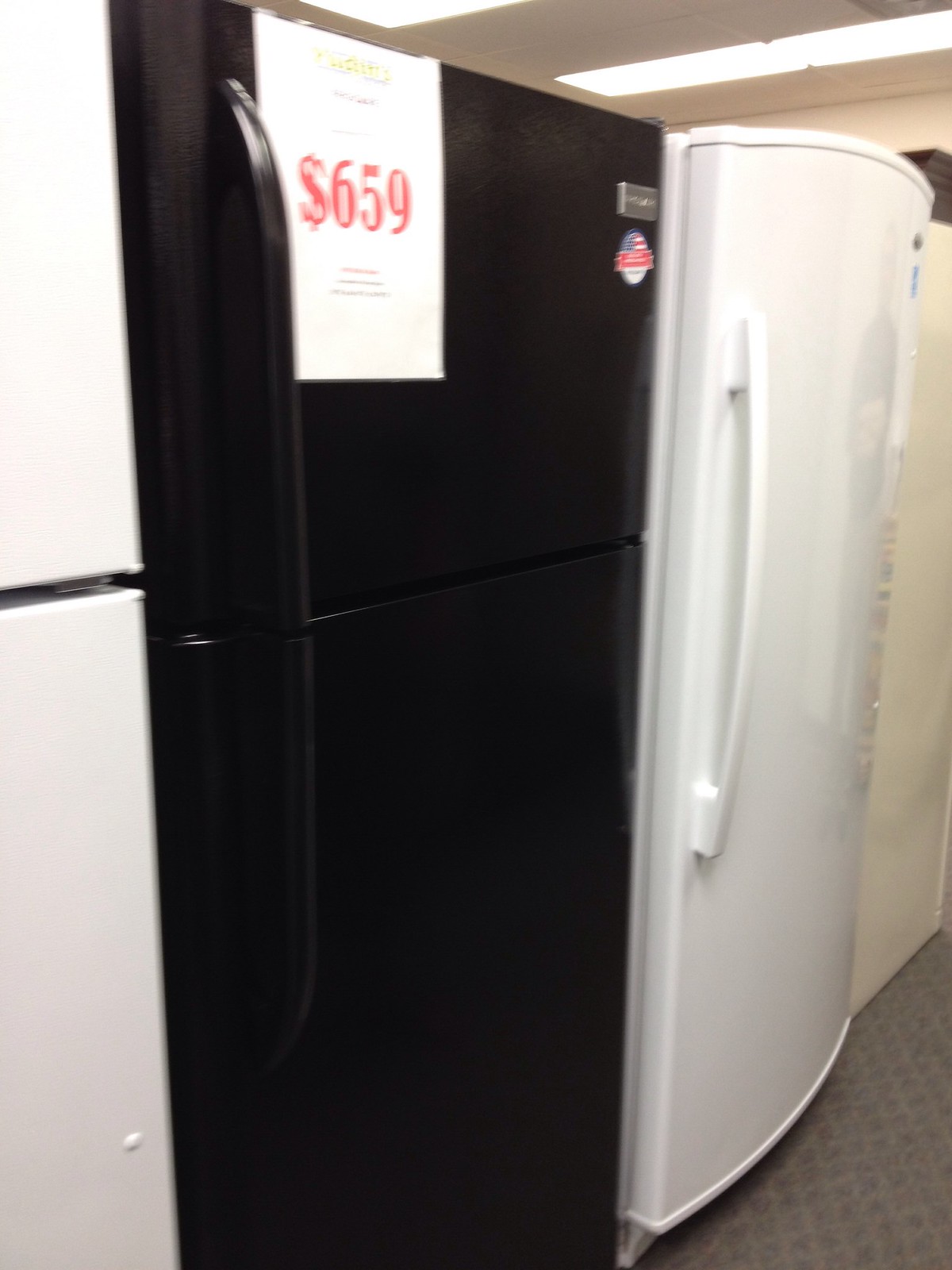In this picture taken inside a store, we see an array of refrigerators on display, illuminated by fluorescent ceiling lights. The floor is covered with a gray carpet featuring subtle square or diamond patterns. On the left side of the image, we can observe a partial view of a white refrigerator. Adjacent to it in the center stands a black refrigerator with a freezer compartment on top and a fridge section below. It features a brand name and a small gray piece of metal in the upper right corner, alongside a sticker and a white piece of paper that prominently displays "$659" in red. On the right side of the black refrigerator, there's another white refrigerator with a single, long door and an elongated handle extending from the top to the bottom. This white refrigerator lacks any additional visible characteristics. The overall scene, complete with the recessed lighting and patterned carpet, clearly indicates it's within a retail environment showcasing these appliances for sale.